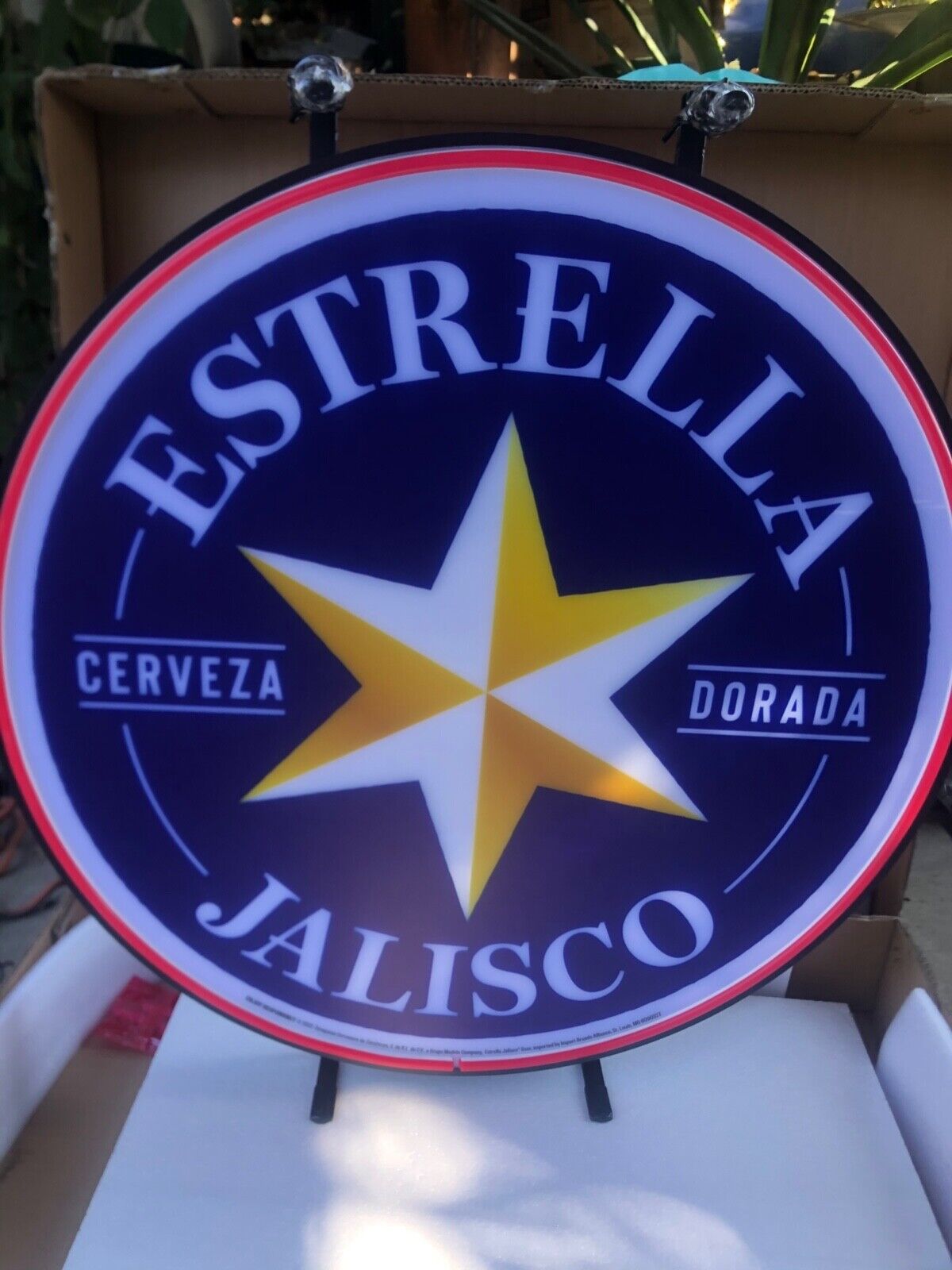The image showcases a circular sign, possibly in its original packaging, which takes up most of the frame. This sign appears to be ready for mounting or hanging. The sign features a multi-layered border, with an outermost circle of red, followed by a gray circle, and then a dark background. In the center, there is a distinctive six-pointed star, with each point bisected by a line, creating an alternating color pattern of white and yellow for the left and right halves, respectively. The star stands out against a blue field, which bears white lettering that reads "Estrella Jalisco Cerveza Dorada." This is a trademark sign for the brand "Estrella Jalisco," a Spanish phrase meaning "Star" and referring to a type of beer. The background also includes boxes, suggesting the sign has just been unboxed, and it is mounted with two clear thumbtacks.